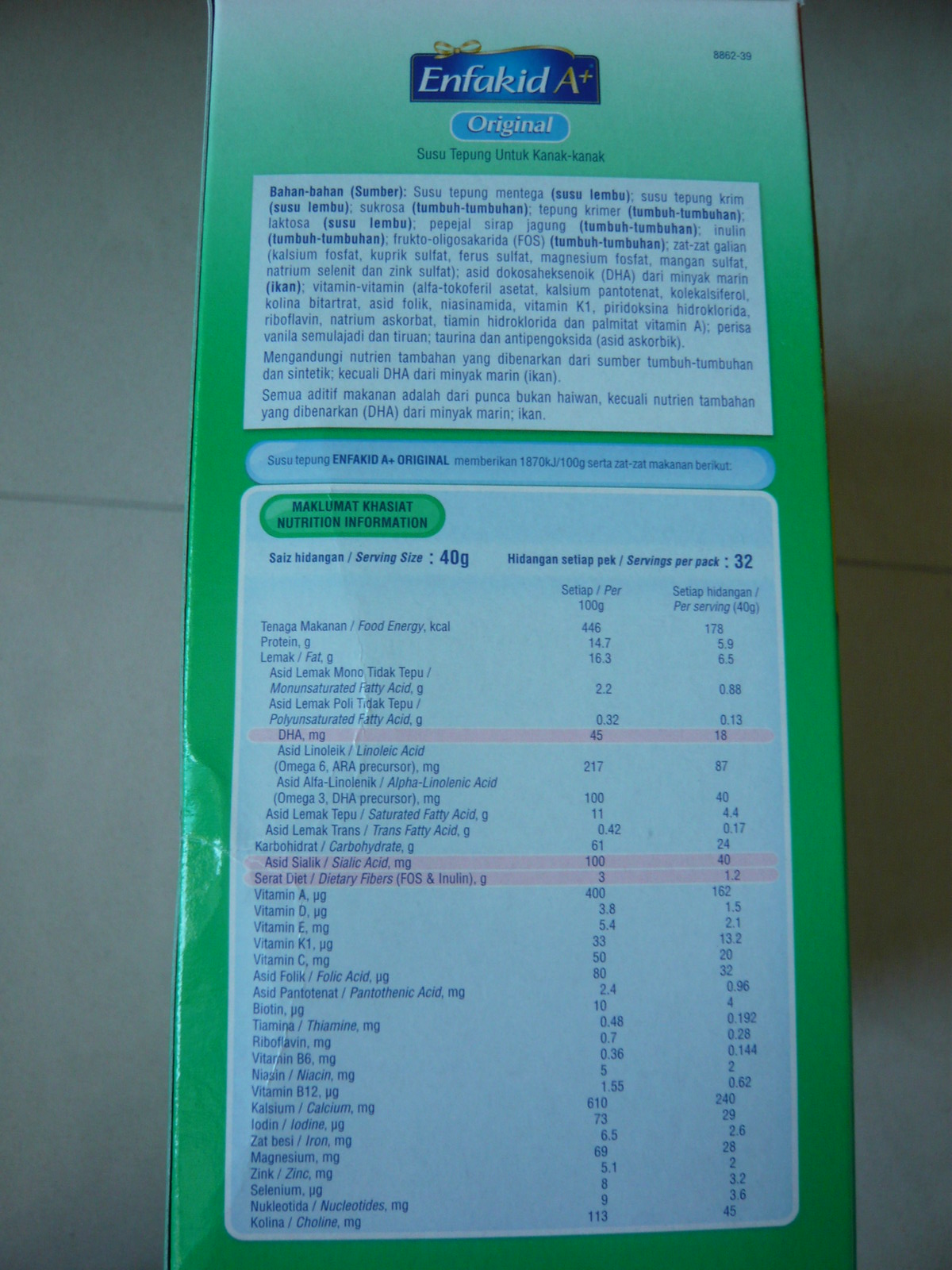The back of the Enfa-Kid Original A+ carton prominently features the brand name "Enfa-Kid" in bold blue letters, accompanied by the "A+" symbol in vibrant gold. The carton is primarily green, enhancing its visual appeal, with a distinct green-highlighted area at the bottom. This area is somewhat difficult to decipher due to its small size. The top section of the carton meticulously lists the ingredients and their respective benefits, particularly highlighting essential vitamins. The labels are crisp white with clear blue text, detailing the nutritional information and benefits concisely.